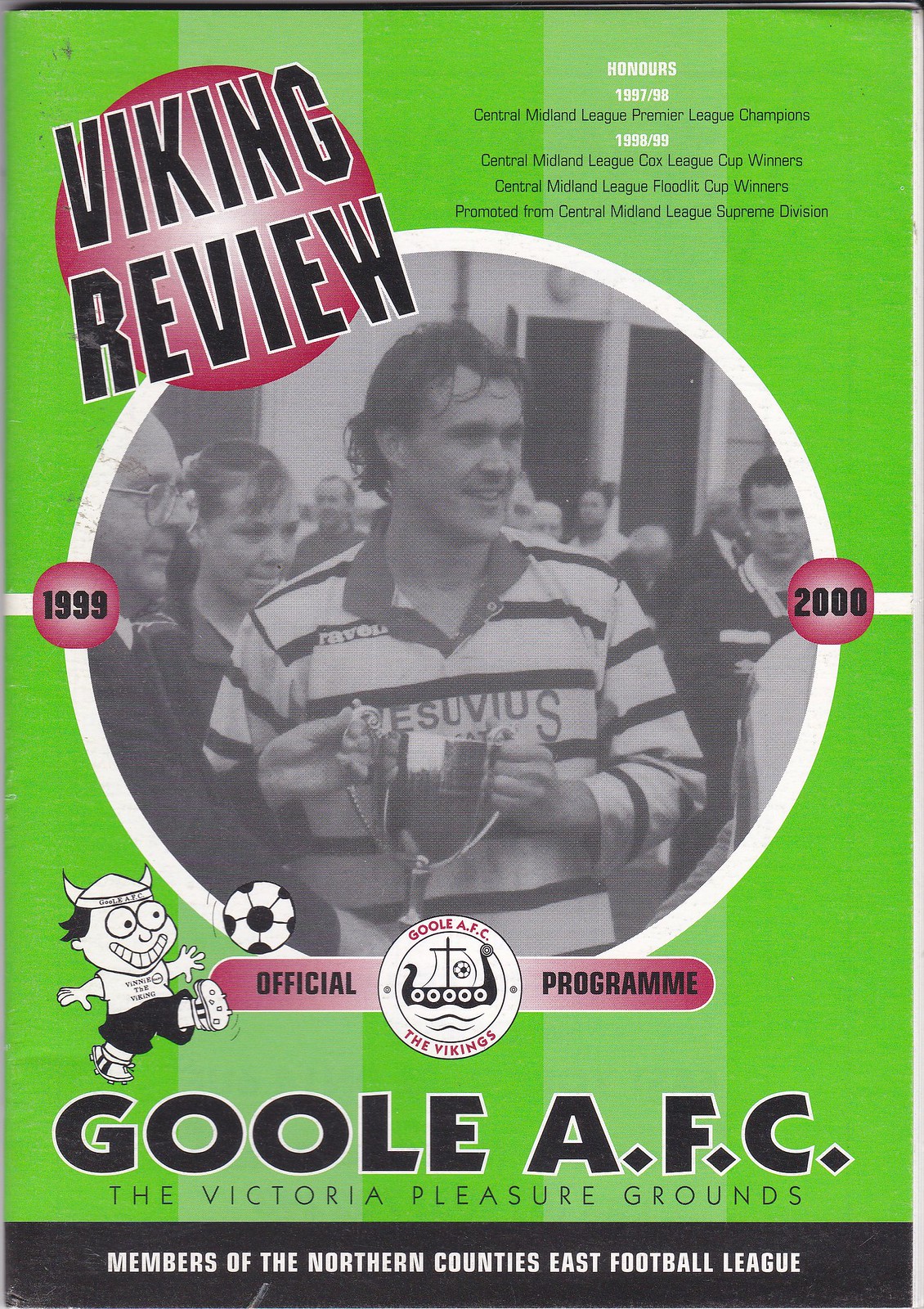The image showcases the cover of an official soccer program with a vivid lime green background that prominently features various elements. At the top left, a pink circle highlights the title "Viking Review" in bold black letters. Central to the design is a black-and-white photograph of a man with long hair wearing a striped long-sleeve shirt, holding a small cup-style trophy. This photograph is encircled by a white border. Surrounding the man, though less distinct, are other people including a person with glasses on the left and a woman on the right. Flanking the photograph are the years "1999" on the left and "2000" on the right. Beneath the central image, black text reads "Official Program." Further down in large black letters, "GOOLE A.F.C. The Victoria Pleasure Grounds" is prominently displayed. Below this, a cartoon figure wearing a Viking helmet kicks a soccer ball into the air. At the very bottom, a black strip with white lettering declares the club as "Members of the Northern Counties East Football League." Additional accolades in white font, such as "Central Midland League, Premier League Champions," and "Central Midland League Floodlit Cup Winners," honor the team's achievements from "1997 to 98" and "1998 to 99."